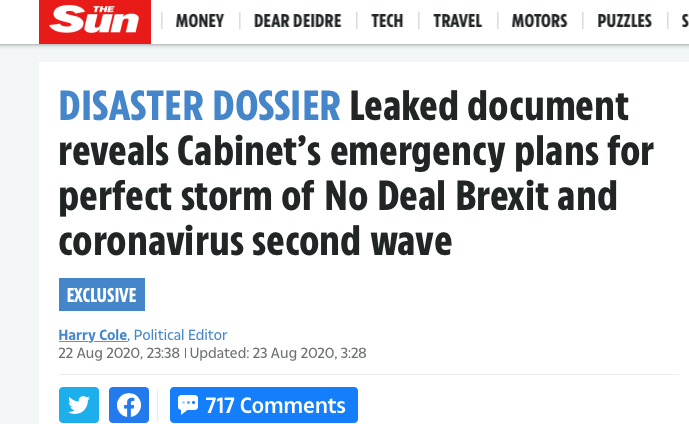In this image, a variety of interconnected categories are prominently showcased against a stark white background. The categories include 'The Sun,' 'Money,' 'Dear Diary,' 'Tech,' 'Travel,' 'Mortals,' 'Puzzles,' 'Disaster Dosia,' 'Leaked Documents,' 'Reveals,' 'Cabinet Emergency Plan for Perfect Storm of No Deal Brexit and Coronavirus Second Wave,' 'Exclusive,' and 'Harry Kohl, Political Editor.' The image also displays a timestamp: Date - 22 August 2020 at 11:38 PM, updated on 23 August 2020 at 3:28 AM. Additionally, social media platforms 'Twitter' and 'Facebook' are listed, accompanied by '717 News' and 'Colosia' in vibrant hues of red, blue, and black. These elements are set in a minimalist layout, with no other details to distract from the primary focus on the listed categories and timestamps.